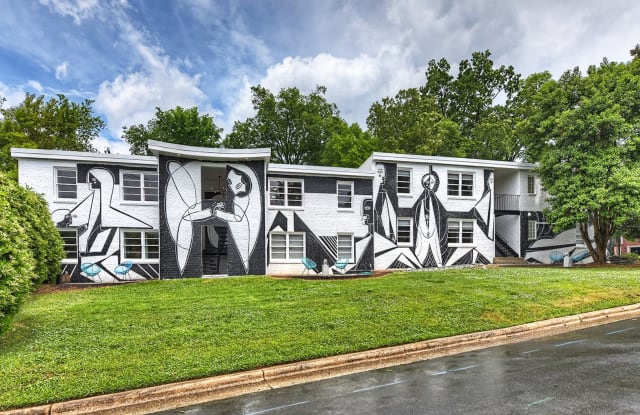The image shows a two-story residential building, possibly an apartment complex, with a striking black and white exterior. This building stands out due to its intricate abstract designs, reminiscent of Salvador Dali or Picasso, featuring human-like and animal-like shapes. The art gives the facade a very modern, almost surreal look. The building is situated along a street with a well-maintained, dark green grass yard in front, flanked by lighter green bushes on the left and a tree line on the right. There are two stairway entrances, one on the left and one on the right, each leading to the building's interior. Blue wicker chairs add a splash of color and are noticeable in front of one of the houses. Behind the building, green trees rise towards a sky filled with a mix of white clouds and remnants of gray storm clouds. The overall scene is framed by a slightly wet, gray paved road in the foreground, hinting at a recent rain shower. The architectural design, coupled with the vibrant landscaping, creates a unique and visually captivating residential area.